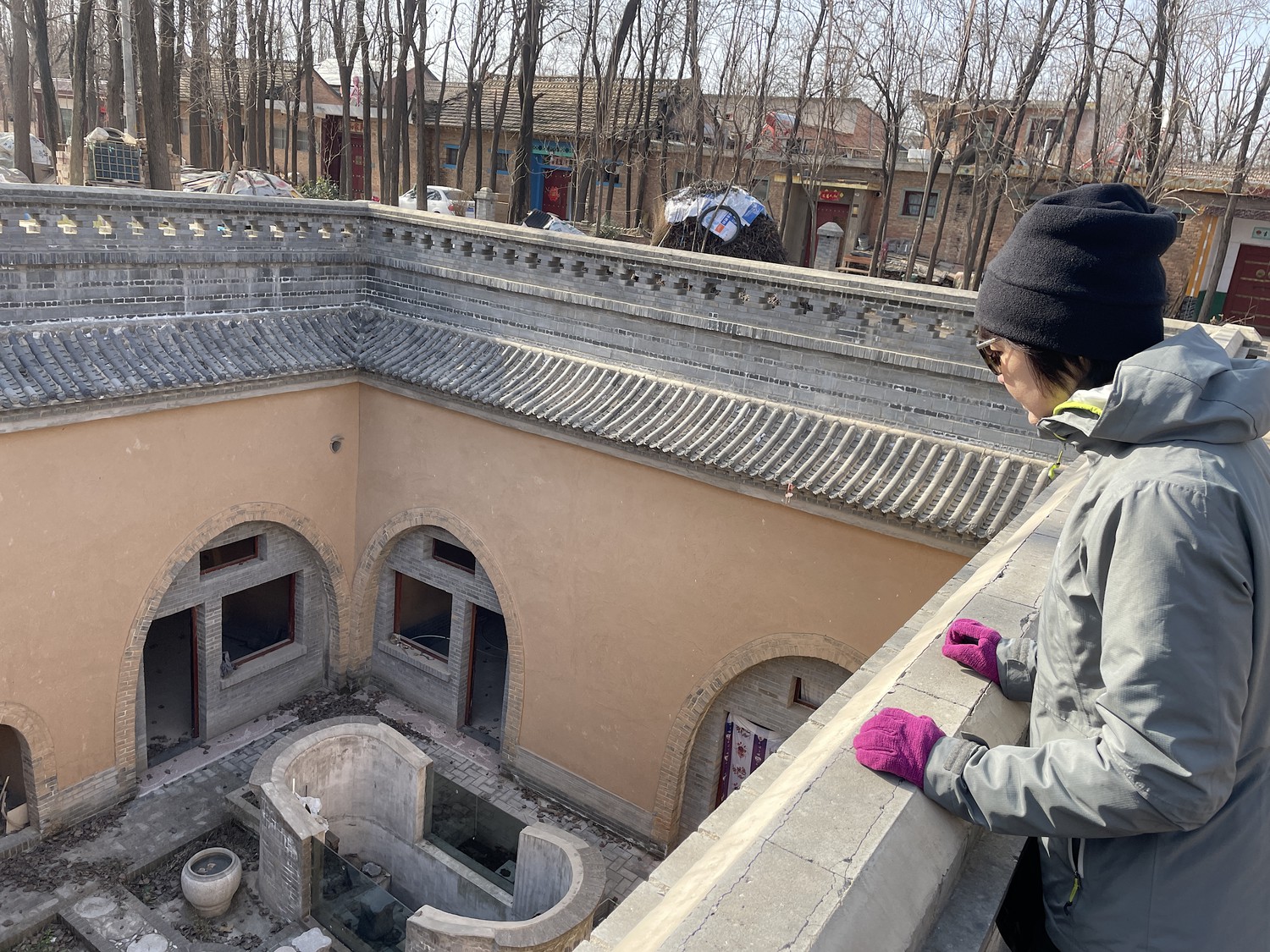In the image, an older, vacant-looking neighborhood, possibly closed down or under renovation, is depicted in what appears to be winter, given the lack of foliage on the numerous trees and the cold weather suggested by the woman's attire. On the right side of the image stands a woman clad in a grey jacket with a hood, a black beanie covering her black hair, purple gloves, and sunglasses. She is gazing down over a stone railing into a dreary residential-type courtyard below. The courtyard's cement floors and beige-painted walls are cluttered with debris and lack doors on their hinges. An old, empty, and degraded hot tub sits among the detritus. Surrounding the courtyard are rows of small, seemingly abandoned shops or buildings, with an overall trashed and neglected appearance. The sky is overcast, amplifying the desolate feel of the scene.